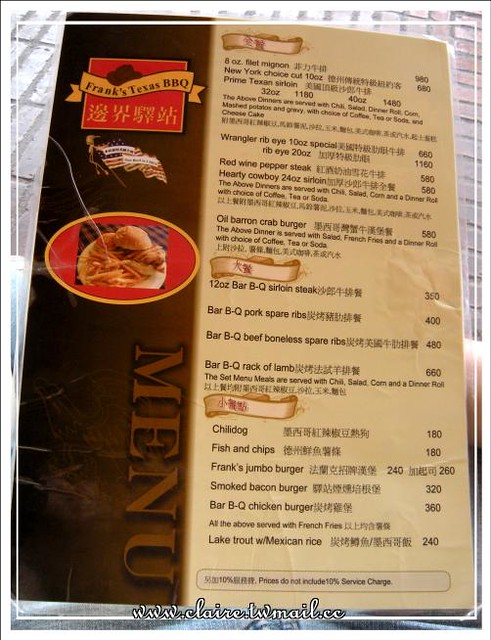The image depicts a brightly lit scene taken during the daytime, as evidenced by the sunlight illuminating the top left and top right corners. Dominating the background is an orangeish-red brick wall, which reflects the daylight, enhancing the brightness of the scene. In the bottom middle part of the image, there is a web address displayed in bolded white text with a black outline. It reads "www.claire.pwmail.cc."

The central focus of the image is a large flyer or pamphlet showcasing a restaurant's menu. This menu occupies the majority of the image, approximately 90%-95% of the frame, and is vertically oriented with a long rectangular shape. The menu is divided into two sections: the left section, which constitutes about one-third of the space, and the right section, which takes up the remaining two-thirds.

The left section features a brownish background with the text "Frank's Texas BBQ" prominently displayed at the top, followed by additional text in a foreign language underneath. The right section of the menu showcases various menu items listed against a tannish brown background, written in black text. Some of the menu items include:

- Le Mignon
- New York Choice
- Prime Texas Sirloin
- Wrangler Ribeye
- Red Wine Pepper Steak
- 12oz BBQ Sirloin Steak
- Bar
- BBQ Pork Spare Ribs

The prices for each item are clearly listed on the far right side of this section, making it easy for customers to view their options and associated costs.